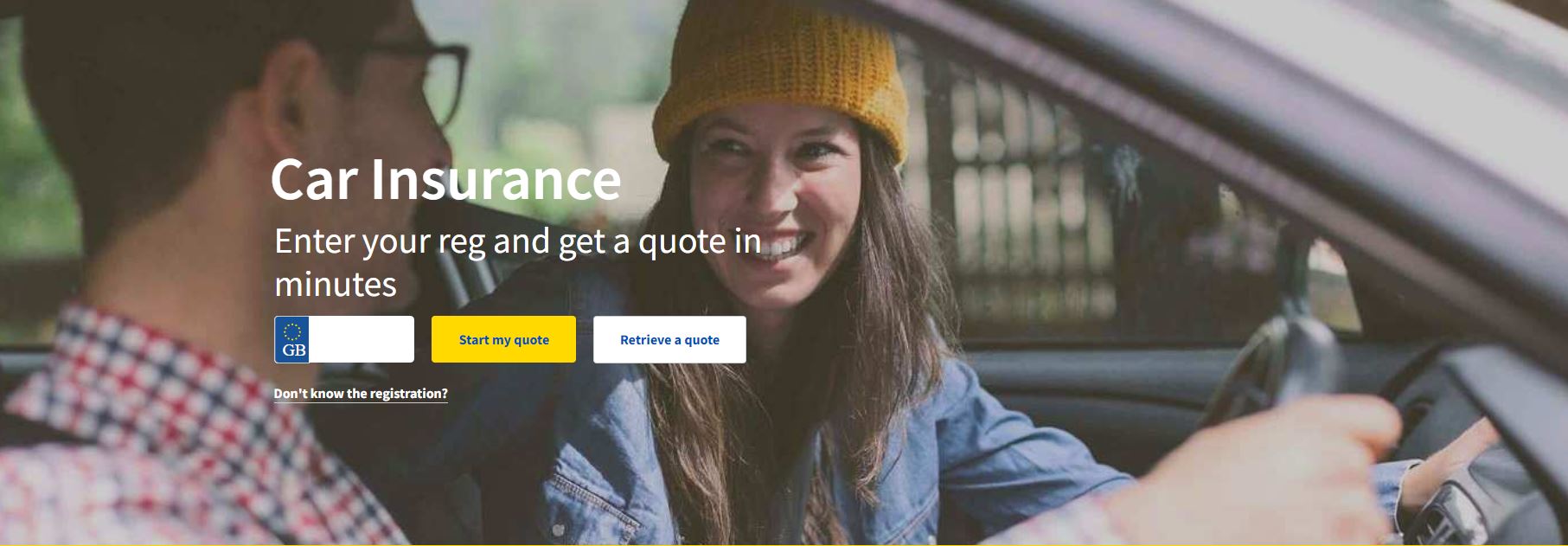A screen capture from an advertisement for a car insurance company, featuring a man and a woman inside a car. The woman, with long brown hair and a cheerful smile, is wearing a yellow beanie and what appears to be a denim jacket. Beside her, the man sports dark sunglasses and has short brown hair, dressed in a red and navy plaid shirt. Both are wearing seatbelts. Overlaid on the image in white text, it reads: "Car Insurance. Enter your reg and get a quote in minutes." Below this, a series of boxes provide interactive options: the first one is white with a blue "GB" and is blank, the second is yellow with blue text that says "Start my quote," and the third is white with blue text that says "Retrieve a quote." There's also a white text line with a question mark that reads: "Don't know the registration?" Through the car window, a black gate and blurred green trees are visible, with sunlight casting a glow on the woman's face, highlighting her bright white teeth. The steering wheel is just visible in the foreground. No other significant objects are notable in the image.